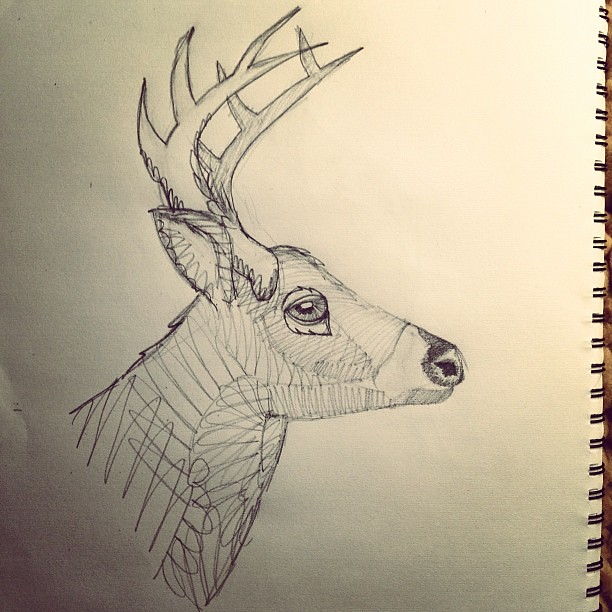The image is a portrait-oriented photo of a spiral-bound artist's notepad, with the spiral binding visible on the far right edge of the frame. The visible portion of the notepad features a meticulous hand-drawn rendering of a deer. The deer is depicted with prominent antlers, each sporting four distinct points. The drawing highlights the deer's expressive, large eye and a prominently black nose. One ear is clearly visible on the right side of the deer's face, adding to the lifelike quality of the illustration. The edges of the notepad are slightly cropped out of the photo, accentuating the artwork's presence within the frame.